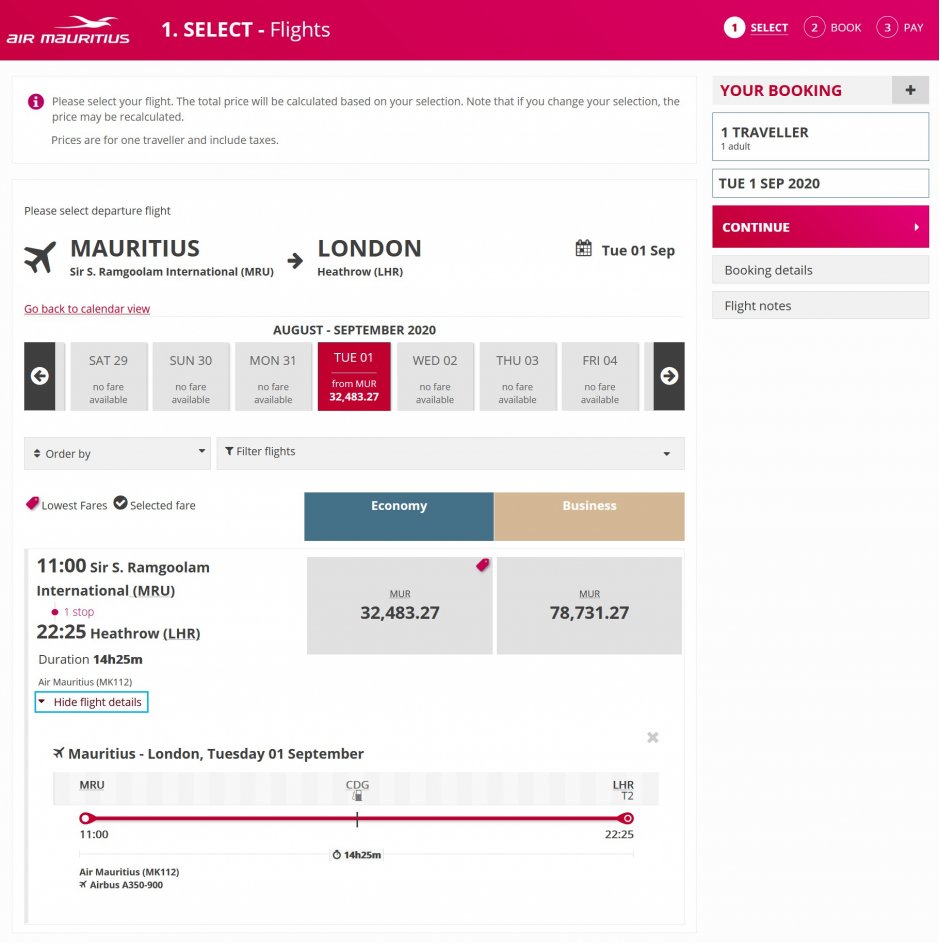The image showcases a flight booking interface for Air Meritus, highlighted in a dark pink colored rectangle at the top left corner. The airline's name is accompanied by a white icon of a flying bird. In the same bar, there is a progress bar indicating steps to select, book, and pay for the flight, with "Select" being highlighted in white, followed by a dot, while "Flights" appears with a capital F.

Centered in this bar is a red circle icon with the number one inside it, followed by steps "Two Book" and "Three Pay," with step one—selecting the flight—currently highlighted.

Below this, there is an instructional text: "Please select your flight. The total price will be calculated based on your selection. Note that if you change your selection, the price may be recalculated. Prices are for one traveler and include taxes."

On the right side of the interface, it displays "1 Traveler, 1 Adult, TUE 1 SEP 2020." Below, there is a pink button saying "Continue" with a right-facing arrow, followed by "Booking Details" and "Flight Notes."

The flight details indicate a journey from Sir Seewoosagur Ramgoolam International Airport (MRU) to London Heathrow (LHR) on Tuesday, 1st September 2020. Additionally, different price fares for various days of the week are visible, with the selected option highlighted.